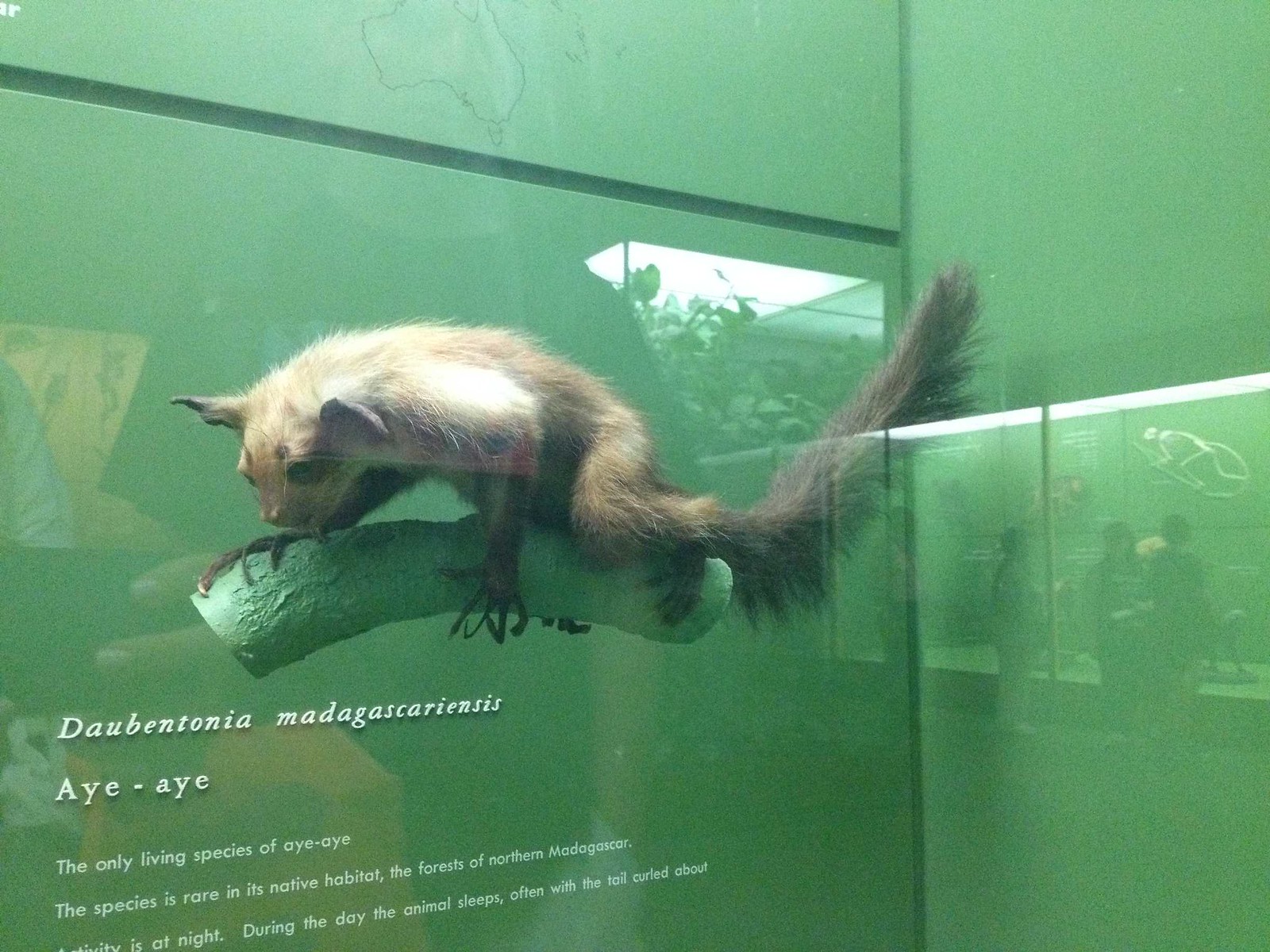The image depicts a zoo exhibit featuring an aye-aye (Daubentonia madagascariensis) in a glass enclosure. The background is dominated by green walls and a white branch against which the animal is perched. The aye-aye has distinctively long fingers, a tiny body, a tiny head with large ears, and a dark, bushy, brown tail. Reflections on the glass enclosure reveal the exhibit's setting, with hints of other enclosures and visitors. White lettering in the bottom left provides informational text: "Daubentonia madagascarensis," "aye-aye," and details about the animal being the only living species of aye-aye, which is rare in its native habitat—the forests of northern Madagascar. The text mentions that the aye-aye typically sleeps during the day, often with its tail curled about. The animal's fur color is a combination of brown, tan, and dark brown, contributing to its exotic and intriguing appearance.